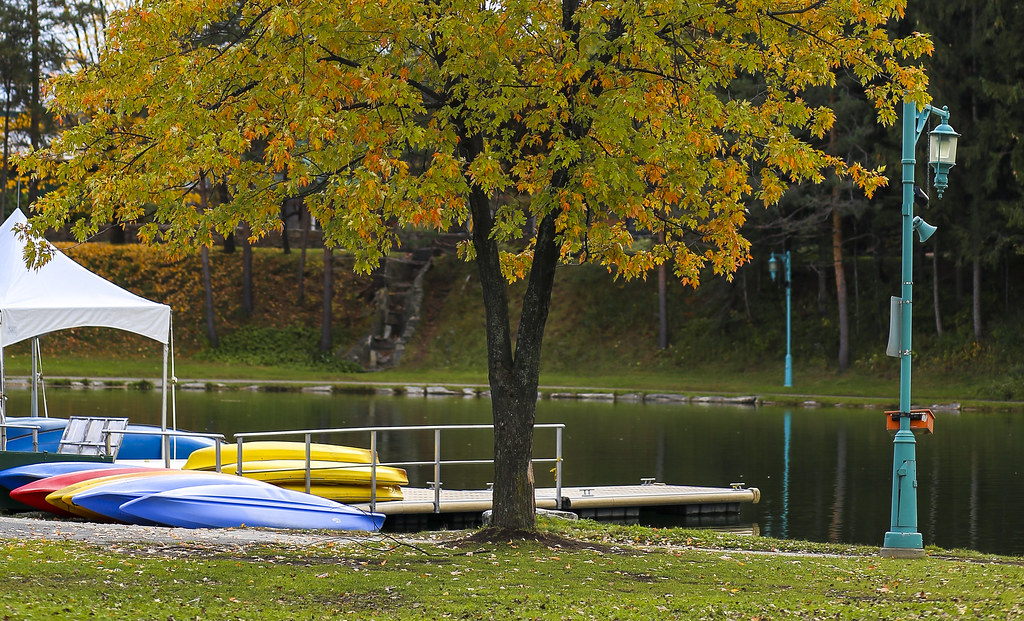This outdoor photograph captures a serene riverside scene. In the foreground, a tree with a distinctive V-shaped trunk stands prominently, its foliage a mix of green and orange leaves, signaling the arrival of autumn. On the riverbank closest to the camera, a small pontoon or jetty with a metal guard rail extends into the water. Several colorful canoes are turned upside down nearby, including blue, yellow, and red ones. Adjacent to these canoes is a tent with a white cloth covering, adding a rustic touch to the scene.

To the left of the tree trunk are the jetty and canoes, while to the right stands a turquoise metal street lamp. The lamp features a hanging lantern suspended from a bracket, adding a quaint charm to the setting.

Across the river, the opposite bank is lined with similar slender trees, their trunks rising to support canopies of green leaves. The overall composition of the photograph evokes a peaceful, autumnal atmosphere, with the calm river reflecting the tranquil environment.